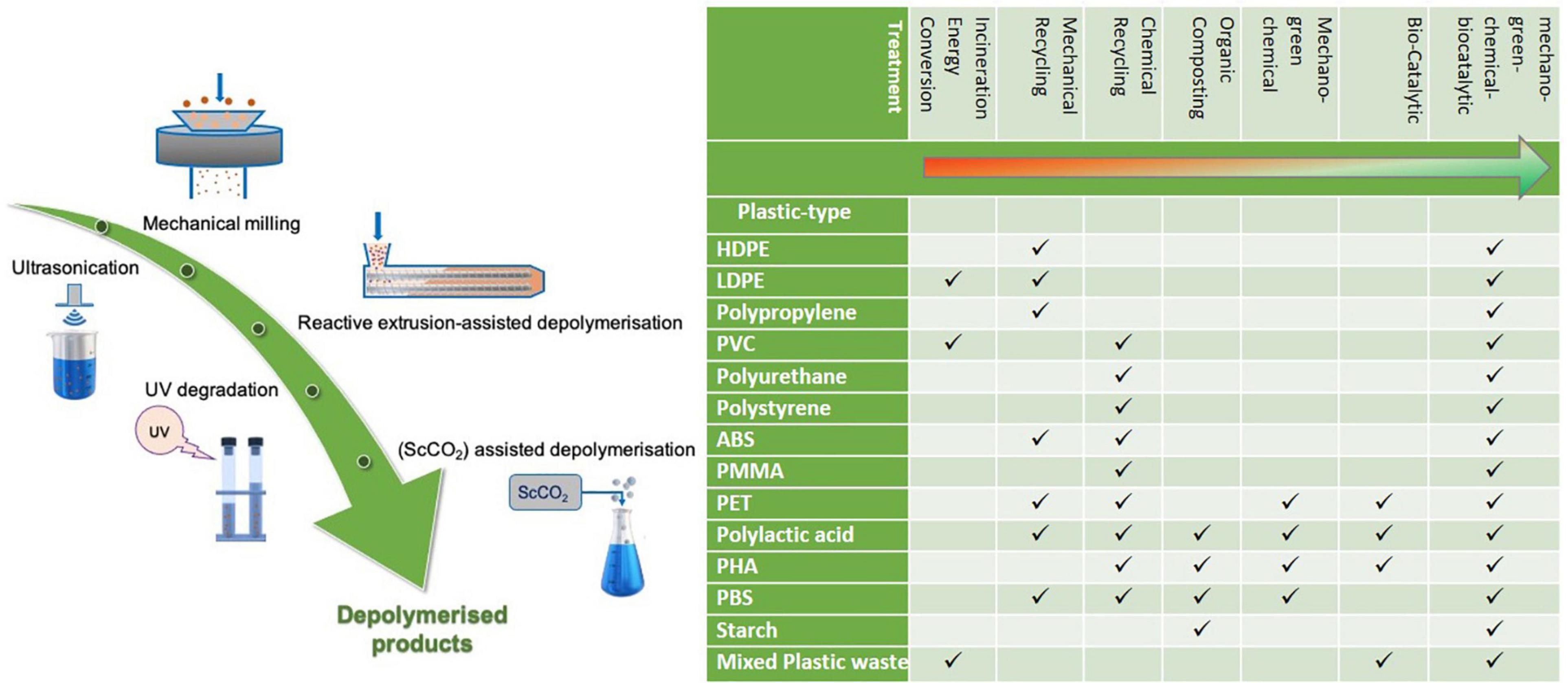The illustrated image is a detailed full-page representation, likely from a science textbook, demonstrating the stages and treatments in a polymerization or depolymerization process. On the right-hand side of the image, there is a color-coded chart in varying shades of green. The vertical axis of this chart is labeled "Plastic Type," listing different types of plastics, while the horizontal axis is titled "Treatment," indicating various treatments such as biocatalytic, mechanical, green chemical, organic composting, chemical recycling, mechanical recycling, incineration energy conversion, and others. The treatments are marked with check marks under the relevant plastic types.

To the left of the chart, there are detailed illustrations depicting various stages of the chemical process involved in depolymerization. These include mechanical milling, ultrasonification, reactive extrusion-assisted depolymerization, and UV degradation, with further details such as CSCO2-assisted depolymerization. The illustrations incorporate visual elements like blue tubes filled with chemicals, images of scientific equipment, and orange materials composed of tiny balls. Additionally, an arrow transitioning from red to green runs beneath these depolymerization stages, with labels like "Ultrasonification" and "UV Degradation" positioned along it. The entire representation is designed to be visually informative and educational, suitable for a scientific context.